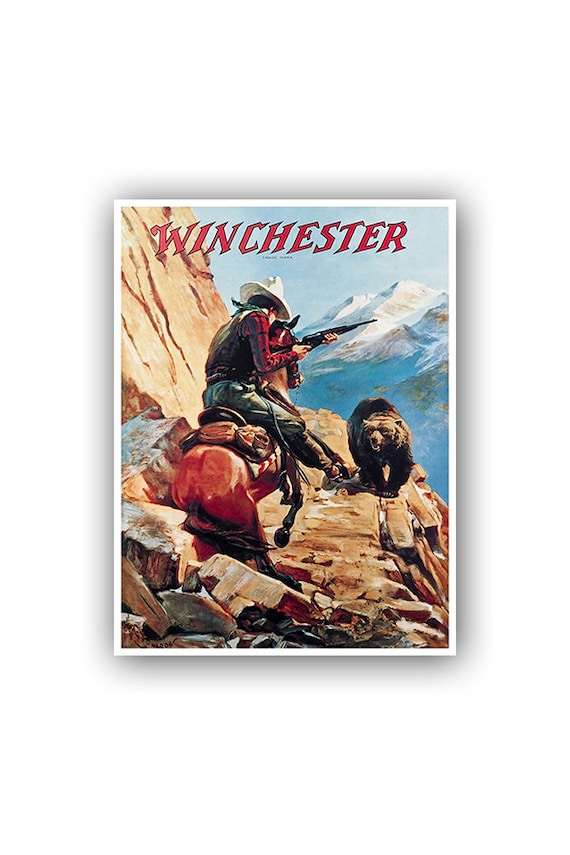The poster, an old advertisement for Winchester rifles, features a dramatic mountain scene within a white border. In the foreground, a rugged, rocky cliff leads to a narrow, precarious ledge where a cowboy, clad in traditional Western attire, confronts an oncoming grizzly bear. The cowboy, astride a rearing horse, wears blue jeans, a red flannel shirt, a white cowboy hat, a leather vest, and a bandana around his neck. He grips a black rifle with both hands, poised to take aim at the bear. His packed supplies can be seen strapped to the horse's back. Behind them, the landscape drops off steeply, revealing a stunning backdrop of snow-capped mountains under a clear skyline. At the top of the image, the word "Winchester" is prominently displayed in bold red letters with a dynamic, lightning-style font.